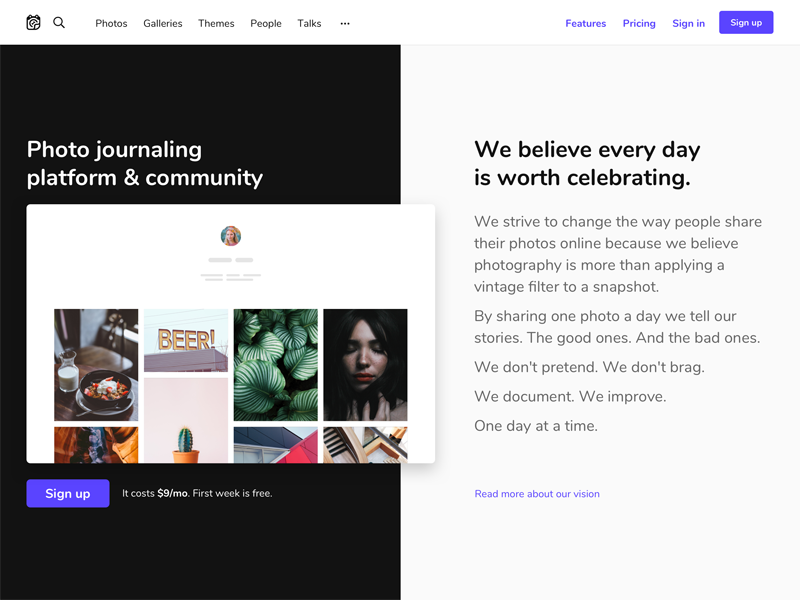**Screenshot Description: Photojournaling Website Home Page**

The screenshot captures the homepage of a photojournaling website on a desktop or laptop computer. The site is dedicated to sharing photos within photojournals, fostering a community of photo enthusiasts.

**Top Navigation Bar:**
- **Left Side:** Features the website logo and a search button.
- **Central Section:** Contains buttons for navigating various sections of the site, including Photos, Galleries, Themes, People, Talks, and a More Options button symbolized by three dots.
- **Right Side:** Provides quick access to Features, Pricing, Sign-In, and Sign-Up buttons.

**Main Content Section:**
The main content area is divided into two parts:
1. **Left Panel:**
   - **Top:** Displays a black background with white text that reads, "Photojournaling Platform and Community."
   - **Below Text:** A sample image gallery showcases what users can build and share on the platform.
   - **Action Button:** A prominent Sign-Up button is highlighted, indicating a subscription cost of $9 per month with the first week free.

2. **Right Panel:** 
   - **Content Block:** Also has a black background but with black text. The text reads: "We believe every day is worth celebrating. We strive to change the way people share their photos online because we believe photography is more than applying a vintage filter to a snapshot. By sharing one photo a day, we tell our stories, the good ones and the bad ones. We don't pretend. We don't brag. We document. We improve one day at a time. Read more about our vision."
   - **Layout:** This content is presented within a square frame for emphasis.

The overall layout and design of the website appear user-friendly, encouraging visitors to join a community that values sincere photojournalism over superficial filters.